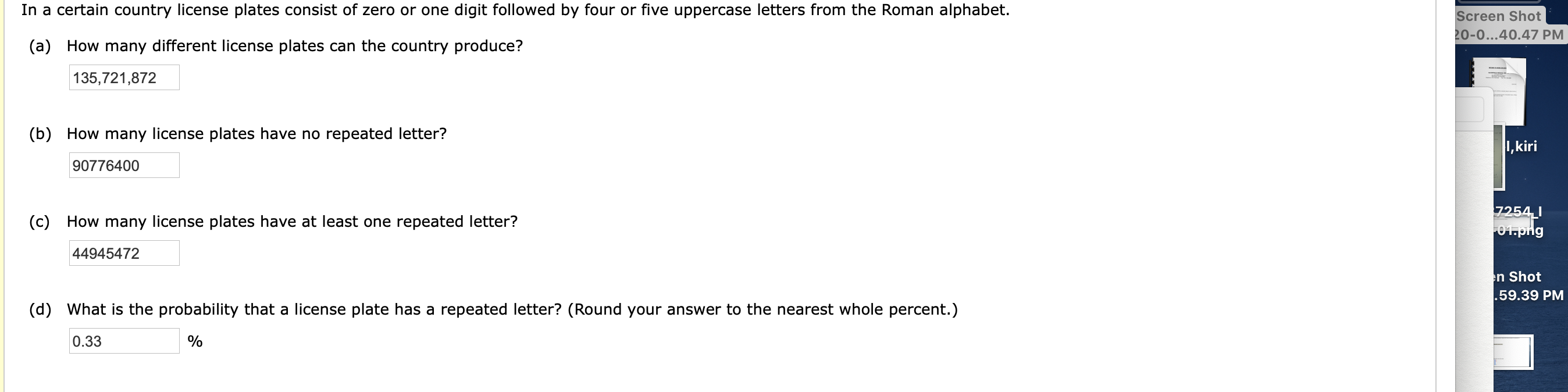This is a detailed screenshot of a test or a series of questions and answers displayed on a white background. The page consists of four questions, each accompanied by a typed response in text boxes below the questions. The print is small and in black. A thin, vertical yellow line on the left side of the page serves as a divider. 

The heading at the top reads: "In a certain country, license plates consist of zero or one digit followed by four or five uppercase letters from the Roman alphabet."

The four questions and their responses are as follows:

1. **Question:** How many different license plates can the country produce?
   - **Answer:** 135,721,872

2. **Question:** How many license plates have no repeated letter?
   - **Answer:** 90,776,400

3. **Question:** How many license plates have at least one repeated letter?
   - **Answer:** 44,945,472

4. **Question:** What is the probability that a license plate has a repeated letter? Round your answer to the nearest whole percent.
   - **Answer:** 0.33%

This structured format clearly presents the information derived from the set of questions and their corresponding answers in a concise manner.